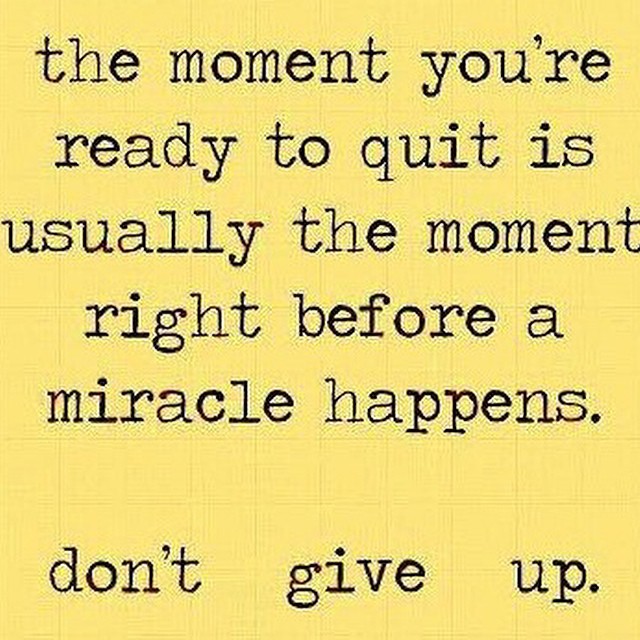The image features an inspirational quote displayed on a bright, yellow background that resembles a piece of grid paper. The paper has faint grid marks, giving it a slightly grainy appearance. In black, grainy typewriter-style text, the quote reads, "the moment you are ready to quit is usually the moment right before a miracle happens. Don't give up." Notably, the text is entirely in lowercase letters. The final three words, "don't give up," are spaced out along the bottom of the image, emphasizing the motivational message. The image is designed as a social media meme, likely intended to inspire individuals who might be feeling discouraged.